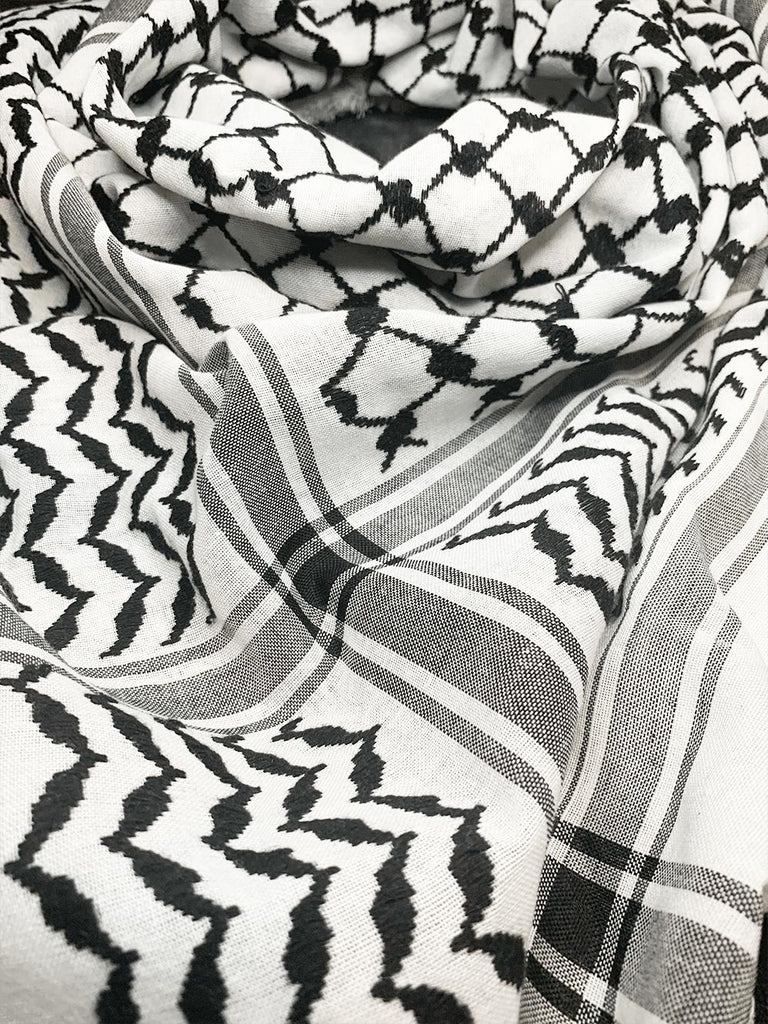The image features a scarf with a detailed and intricate checkered design, reminiscent of traditional Middle Eastern patterns, possibly similar to those found in Palestine or some Muslim countries. The scarf, primarily composed of black, white, and grey elements, features a series of intersecting black lines forming a grid. Some intersections are darker, creating bold black squares. Within the grid, various smaller patterns emerge, including zigzag lines and shapes that resemble barbed wire or squares with dots at the corners, giving the design a somewhat textured appearance. The scarf itself appears to be folded and wrinkled, lying flat on an unseen surface with no additional background elements to provide size context.